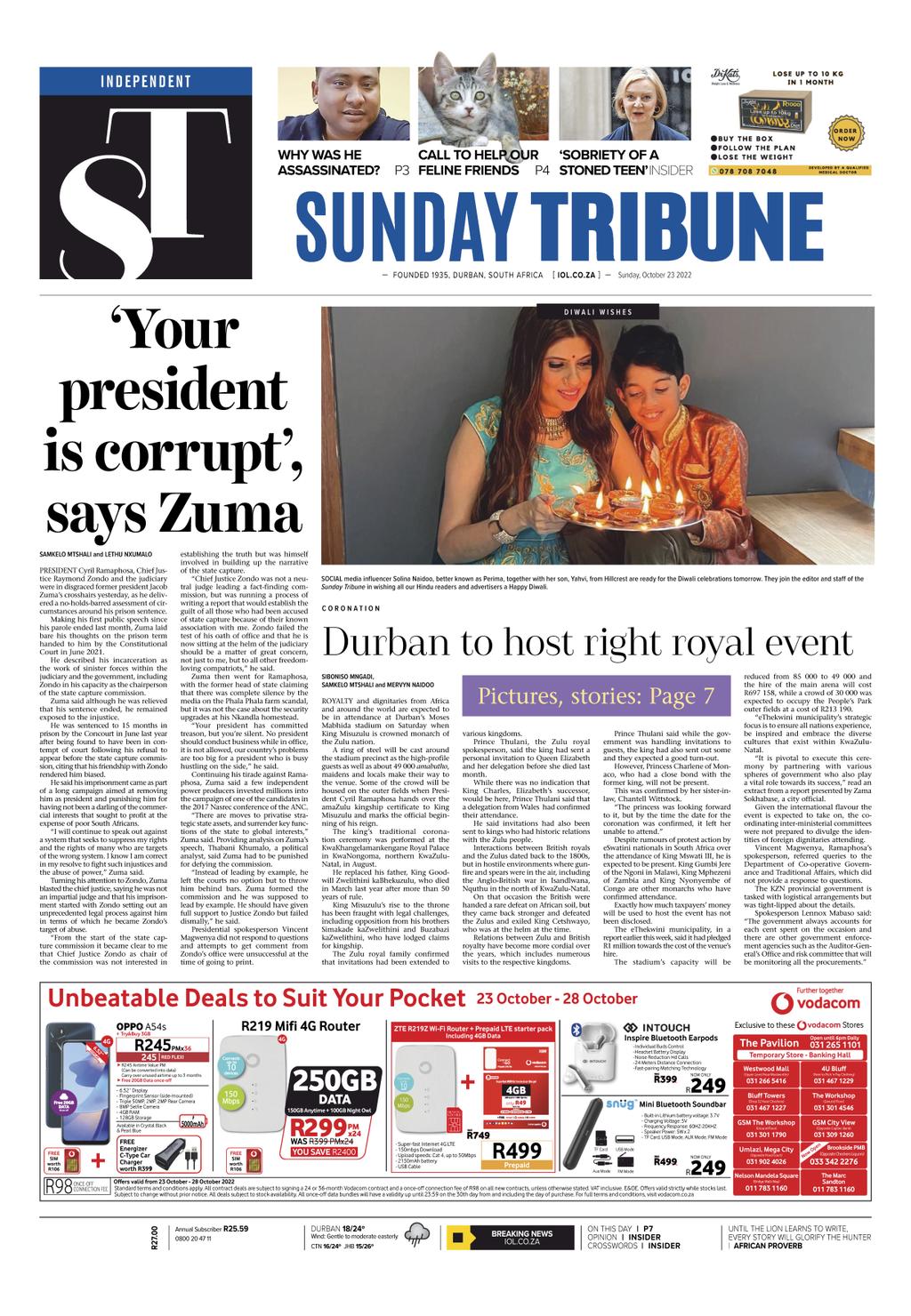On a newspaper website, the left-hand side features a blue rectangle with the word "Independent" and a darker rectangle below it containing the letters "ST." Progressing to the right, there are four images: a man, a cat, a woman, and a box, all accompanied by unreadable captions. Prominently displayed in large blue letters is the title "Sunday Tribune." Below a gray line, a headline reads, "Your president is corrupt," says Zuma. Below this, a photograph of two women holding what appears to be a plate with candles is accompanied by the headline, "Durban to host royal event," followed by text that is too small to decipher. To the right, a purple rectangle with yellow text states, "Pictures, Stories: Page Seven." Further down the page, a gray-outlined rectangle promotes "Unbelievable deals to suit your pocket, 23 October through 28 October," with numerous advertisements below. At the bottom, small, unreadable paragraphs and additional gray lines with more indistinguishable words and symbols appear.